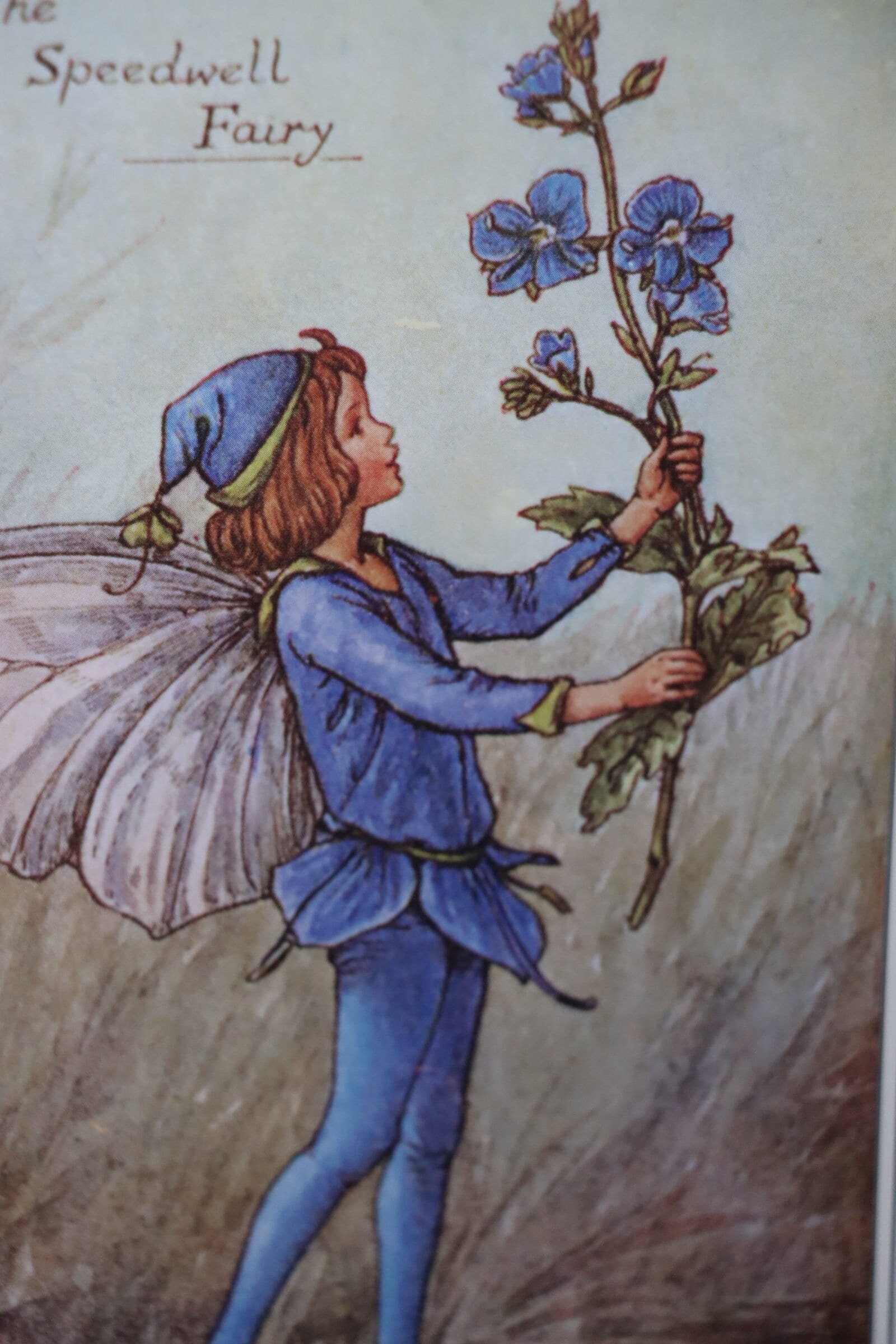The image, titled "Speedwell Fairy," prominently displays this title in underlined brown text in the upper left corner. The artwork is presented in a portrait layout. Central to the image is a fairy child characterized by long brown hair, a blue and green hat resembling a nightcap with a four-leaf clover at its tip, and white, butterfly-like wings attached to its back. The fairy is dressed in a blue outfit, consisting of a shirt that flares out at the waist in the shape of petals and blue tights. The waist is cinched with a green string, matching the trim on the hat and shirt. The child is depicted holding a long-stemmed plant with green leaves and blue flowers, mirroring the colors of its attire. The fairy's demeanor suggests it is gazing up at the plant thoughtfully. The background is a gradient of light blue sky in the upper half, transitioning to abstract patterns of greens and browns towards the bottom, symbolizing grass. The overall setting has a delicate, hand-drawn feel, enhancing the whimsical nature of the fairy and its natural surroundings.